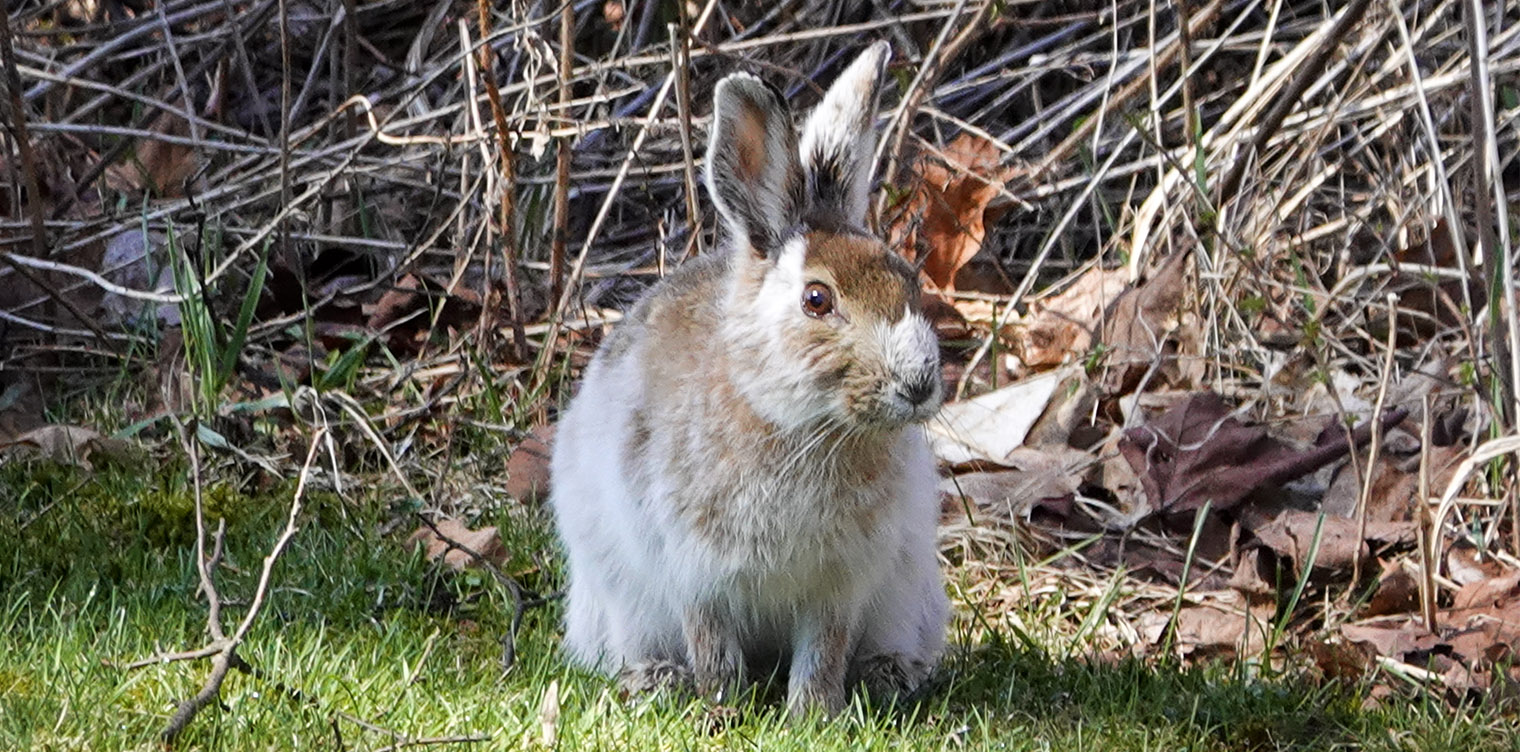This detailed photograph captures a calico-patterned rabbit situated outdoors, centered amidst a vibrant patch of green grass. The rabbit's small feet are hidden by the grass, but its upper body is fully visible, revealing a striking coat of white interspersed with light and dark brown markings. Its dark, alert eyes and a petite black nose add to its expressive face, framed by brown fur between the eyes and a lighter muzzle. The tall ears, white with dark brown at the base and pink interiors, stand erect and slightly angled as if the rabbit has detected a subtle sound. 

The backdrop consists of a mixture of dead leaves, sturdy old weeds, and stick-like reeds, likely hinting at a fall setting given their brown, lifeless appearance. This naturalistically styled setting might be the edge of someone's yard, adding a layer of context to the rabbit's surroundings. The bunny’s posture suggests attentiveness, as it looks slightly off-camera, mindful of its environment. The predominantly white fur contrasts sharply with the green grass and the earthy tones of the background, making the rabbit's presence the focal point of this picturesque scene.